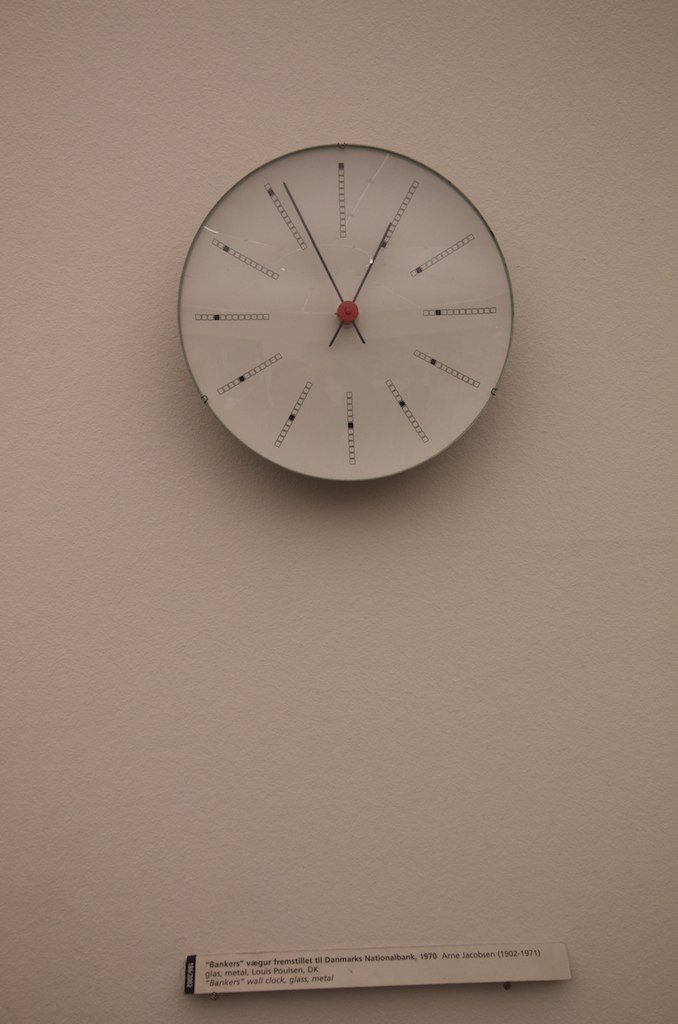The photograph, presented in portrait orientation, captures a white plaster wall with a prominently displayed circular clock central to the top half of the image. The minimalist clock features a slim black trim with a face devoid of traditional numerals. Instead, where each hour would be denoted, there is a vertical row of 12 sections, with the respective section being blacked out to indicate the hour. For example, at one o'clock, the bottom square of the line is shaded. The clock also has slender black hands, indicating the current time is approximately 12:56. Below the clock, about 60 centimeters down, an information label is affixed, likely indicating that this clock is part of an exhibition. The label includes details such as "Bankers' Clock" from Denmark's National Bank, created in 1970 by Jacobsen (1902-1971), and mentions materials like glass and metal. Additionally, the clock appears to have a potential crack in the upper portion of its circle, adding a touch of distinctiveness to this strikingly simple yet unique timepiece.